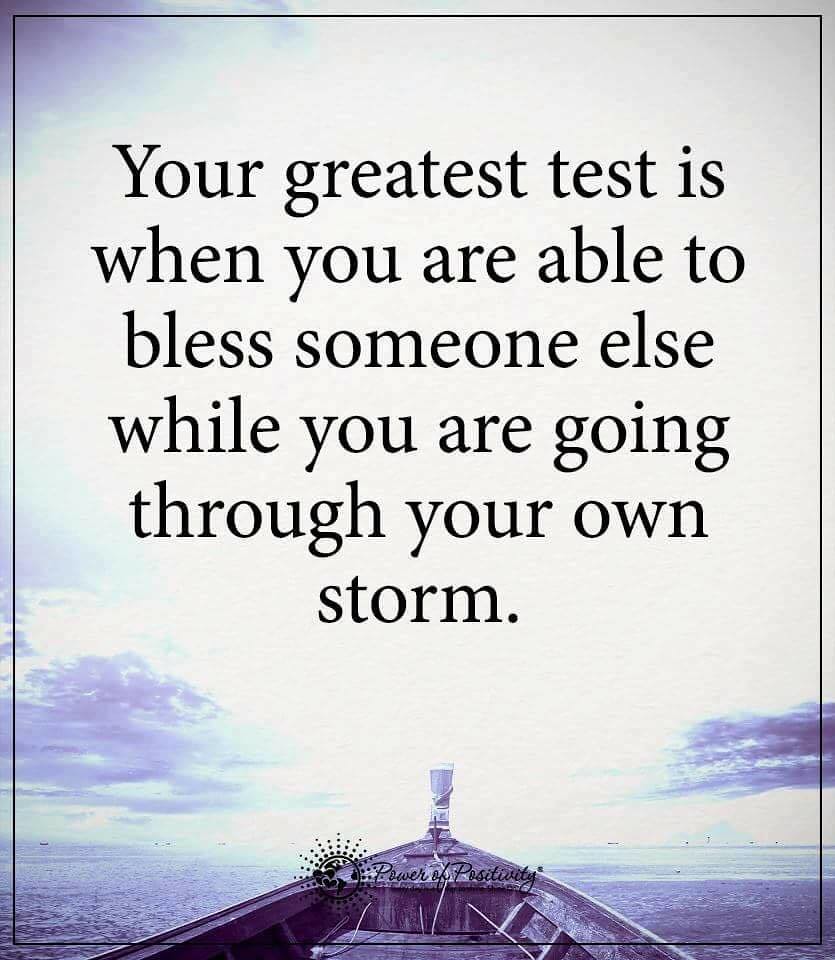This minimalistic, motivational poster features a serene and slightly edited image of an old Viking-style ship sailing through calm waters with a faint sky, tinged with hints of blue, gray, and purple. The scene includes subtle dark clouds on either side, hinting at past or future storms. The main inspirational message, written in bold black text, reads: "Your greatest test is when you are able to bless someone else while you are going through your own storm." Below this, at the tip of the ship's triangular front end, the phrase "Power of Positivity" is inscribed in black ink, accompanied by a globe logo encircled by hearts and radiating dotted beams, symbolizing global positive influence. The entire composition is framed by a thin black line, enhancing its clean and aspirational aesthetic.